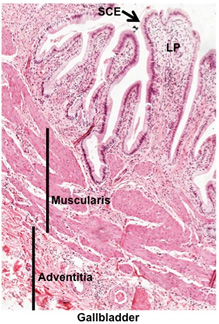The image is a detailed scientific slide depicting a section of human gallbladder tissue, characterized by an array of pink, white, and deep burgundy hues. The intricate patterns and structures visible in the image resemble the view under a microscope. At the bottom, the word "gallbladder" is clearly labeled in black. The tissue is sectioned into different parts: at the lower part, the label "ADVENTITIA" is identified, while above it, the word "MUSCULARIS" is written. In the upper region of the image, the letters "SCE" are indicated by an arrow pointing to an area filled with white, vein-like structures, and nearby the initials "LP" are marked over a pink-speckled region. The overall composition of the image reveals swirling patterns and tubular formations, providing a detailed view of the gallbladder's complex anatomy.